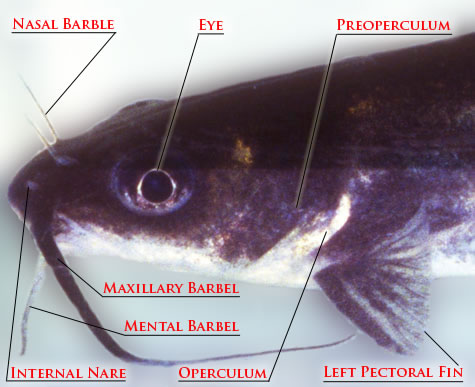This detailed close-up image showcases the left-facing profile of a catfish, highlighting its anatomical features with labeled lines. The fish's body displays a gradient of colors, transitioning from a dark blue-black or purplish back with occasional gold specks, to a silver eye with a prominent black pupil, and further down to a silver or white underbelly. The eye is notably large, drawing immediate attention. Distinctive features such as whisker-like barbels hanging from its face point towards its catfish identity. The labels in red outline various parts: "nasal barbel" at the top left, "eye" with a pointing line, "preoperculum" towards the middle, and "left pectoral fin" at the bottom right. Additional labels include "maxillary barbel," "mental barbel," "internal nare," and "operculum," all meticulously annotated, making this an educational and detailed anatomical illustration of the fish.